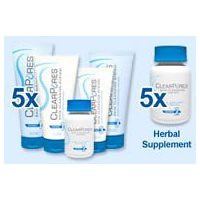The image showcases a detailed advertisement set against a light blue backdrop, promoting an herbal supplement and associated products. Centrally, a white vial with a blue cap, labeled as an herbal supplement, is prominently featured. To its left, there are multiple tubes, apparently of a cream or face wash, also adorned with blue caps. These tubes appear in both white and blue variations, and feature a greenish swirl and some blue lettering. In the foreground, the herbal supplement vial stands out with an enlarged image of it displayed to the side. The text "5X herbal supplement" is highlighted both on the left and right sides of the advertisement, enhancing its visibility. Additionally, the word "clear pores" is mentioned, but with an inverted question mark replacing the 'L' in "places," adding a unique textual element. This advertisement blends the promotion of an herbal supplement with skincare products, all unified by the cohesive light blue background and consistent color scheme in the packaging.